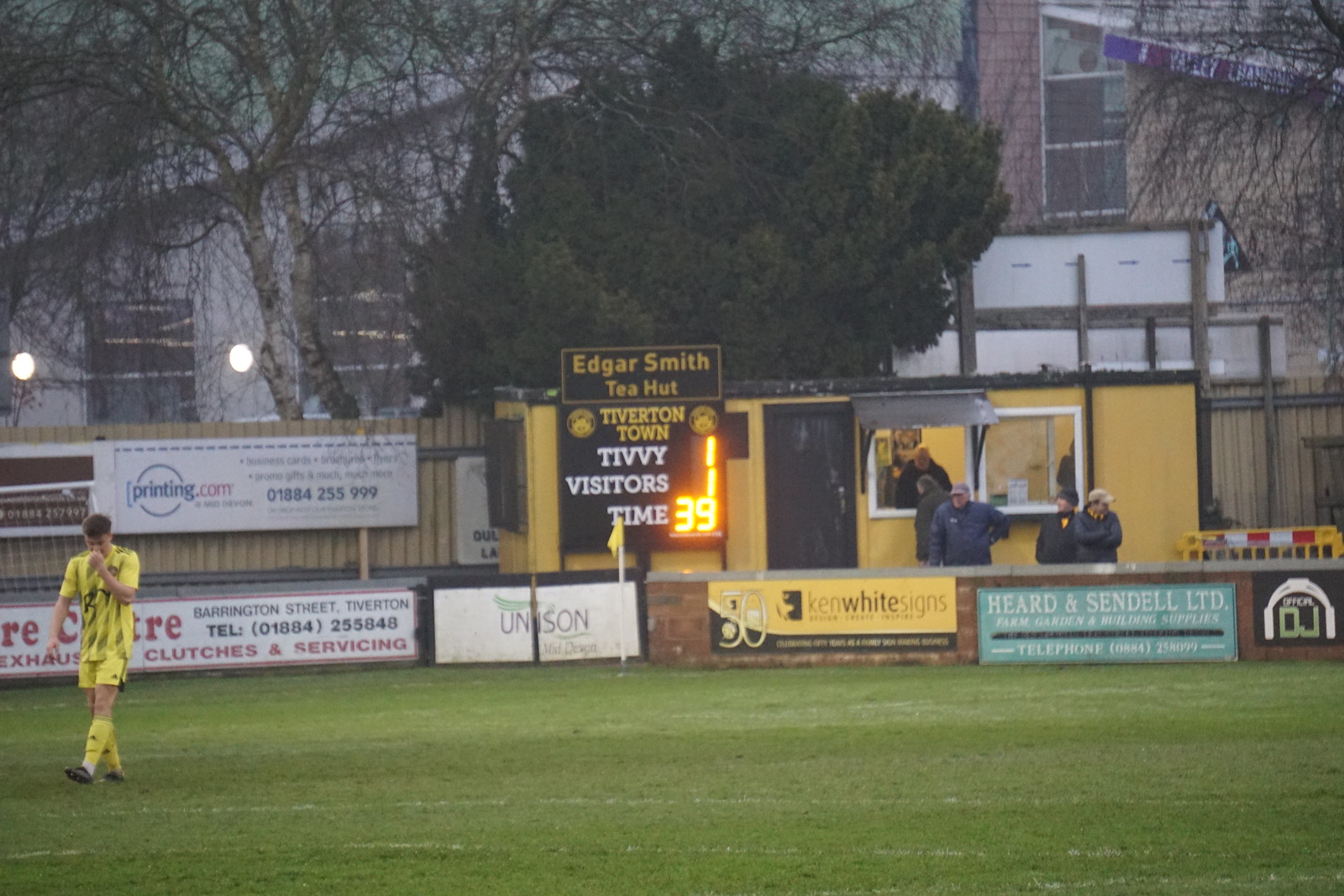In this vivid image taken at a soccer game, the foreground features a lush green soccer field with a lone player sporting a yellow uniform and yellow socks, positioned towards the far left of the field and walking with his head down. The background reveals a bustling scene around a yellow concession stand known as the "Edgar Smith Tea Hut," where people, dressed in coats and hats, are either queuing up or being served tea through its windows. Adjacent to the Tea Hut is a prominent scoreboard displaying "Tiverton Town, Tivy 1, Visitors 1, Time 39," with tall, glowing lights illuminating the field, suggesting it's either late afternoon or early evening. Surrounding the field and the tea hut are numerous advertisements plastered on walls, including "Ken White Signs," "Unison," "Hurd & Sendell Ltd," "Printing.com," along with others promoting local businesses like "Clutches and Servicing," "Farm Garden and Building Supplies," and those featuring phone numbers and addresses like "Barrington Street, Tiverton." To the left of the concession stand is a notable wooden wall with an additional large advertisement for "Printing.com." A tall tree and several buildings form the distant backdrop, conveying a lively community atmosphere at the soccer match.